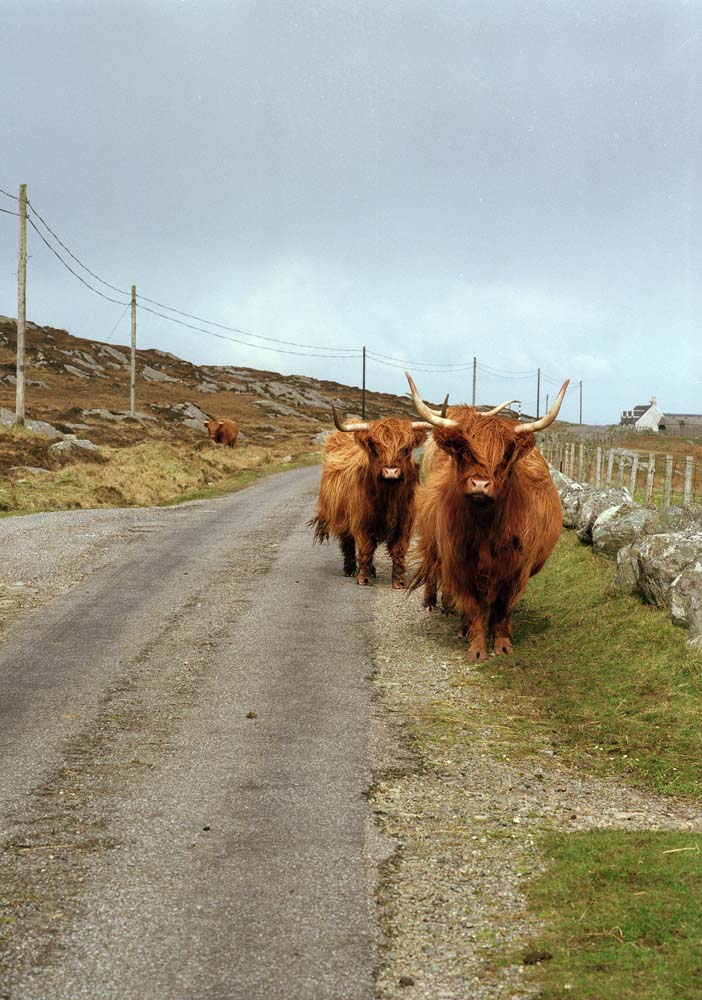In this detailed country scene, three brownish-red yaks with long, shaggy fur and prominent handlebar horns are spotted standing alongside a narrow, concrete road. Two of these majestic creatures are positioned on the right side of the road, close to the foreground, and seem to be looking directly at the camera. The third yak is further back on the left side of the road. The road is bordered by some very short, cropped grass where the yaks are standing and large boulder rocks are scattered nearby. There is a small fence on the right side before these rocks, and a building that could be a house or possibly a barn in the background. Power lines, or perhaps the top of a fence, run along the left side of the road, contributing to the rustic, rocky hillside setting, with gray, cloudy skies above completing the scene. The road appears quite narrow, likely suitable for only one car at a time.